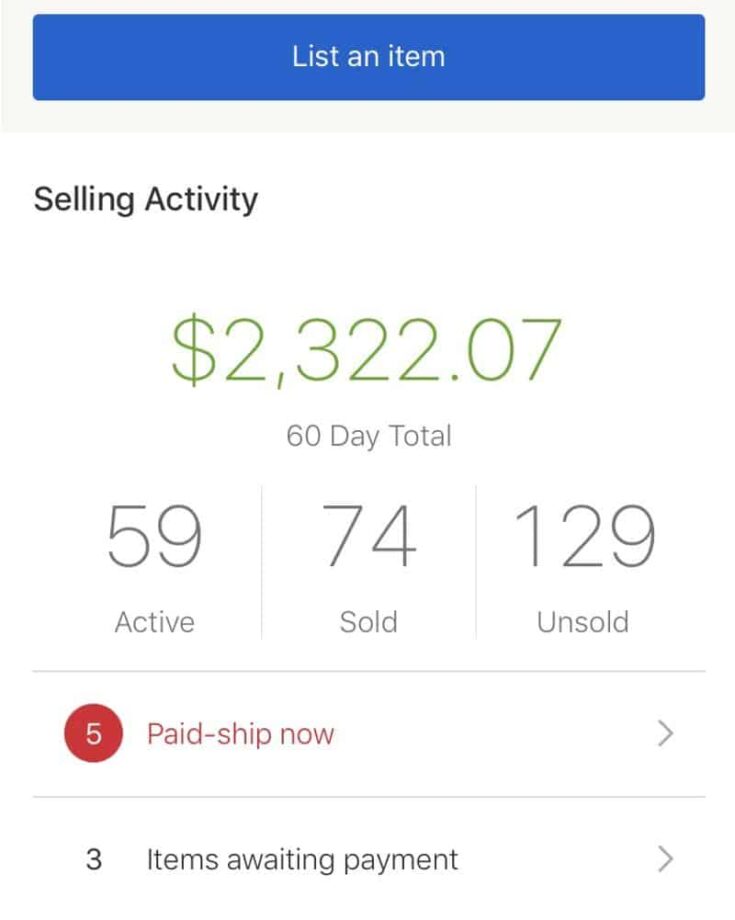The image is a screenshot featuring a clean white background with clearly visible text. At the top of the image, there is a blue banner with white text in the center that reads, "List an Item." Directly below this banner, bold text states "Selling Activity."

Centrally located in the image, large green numerals display a dollar amount of $2,322.07, signifying the 60-day total sales. Smaller black text beneath this amount confirms it as "60-day total."

Further down, there are three categories shown in bold black text, each with accompanying metrics:
- On the left side: "59 active" items.
- In the middle: "74 sold" items.
- On the right side: "129 unsold" items.

In the lower half of the image, a red text banner commands attention with "Paid, Ship Now" alongside a clickable-looking arrow. A red circle with the number "5" to its right indicates items needing shipment. Below this, another segment reads "Items Awaiting Payment," accompanied by the number "3" and another clickable arrow.

This detailed organization aids in efficiently tracking sales activities and actions needed.